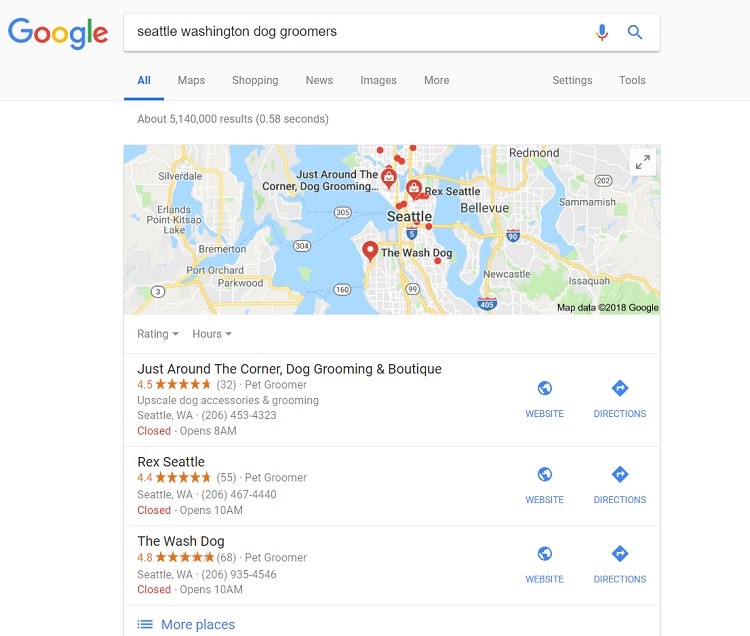The image is a detailed screenshot of a Google search results page. At the top-left, the recognizable Google logo is prominently displayed. Directly to the right lies a search bar containing the query "Seattle, Washington Dog Groomers." Below the search bar, a horizontal menu bar features clickable options: All, Maps, Shopping, News, Images, More, Settings, and Tools. 

Beneath this menu, a clean white space informs the user about approximately 5,140,000 search results, generated in 0.58 seconds. Dominating the top portion of the results page is an embedded map of Seattle, dotted with multiple push pins and red circles indicating various dog grooming locations.

Further below, the first search result highlights “Just Around the Corner Dog Groomer and Boutique,” rated 4.5 stars based on 32 reviews. The text provides additional details: “Upscale Dog Accessories and Grooming, Seattle, Washington,” along with a contact number: 206-453-4323. The listing also specifies that the business opens at 8 am and provides links to its website and directions.

The second result features "Rex Seattle," a pet groomer with a 4.4-star rating from 55 reviews. This entry lists the business as “Pet Groomer, Seattle, Washington,” and includes the contact number 206-467-4440.